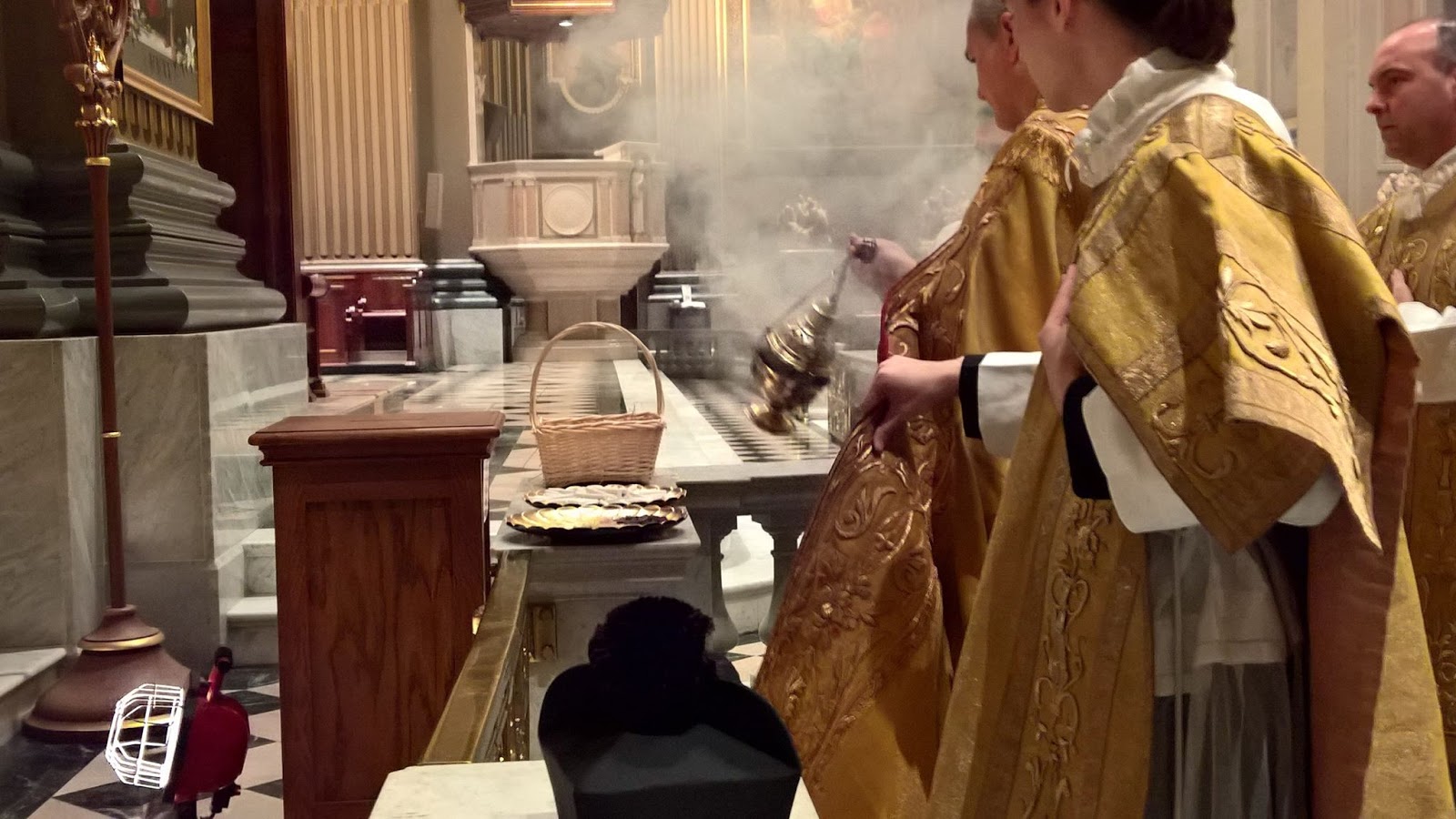In this detailed image of a church service, three men are dressed in ornate, gold ceremonial garments with white collars over their outfits. They stand before the church’s splendid altar, which features a marble wall and checkered tile flooring. The priest, accompanied by an altar boy who is closest to the viewer, is seen mid-motion as he swings a metal censer emitting holy smoke, possibly containing frankincense. The priest blesses part of the altar, while the third figure, whose title is unclear, stands behind them. The space around them is grand, characterized by the large, raised marble podium across the church and a light-colored marble balcony that can be glimpsed through the haze of the smoke. Visible are also a black item on one of the pews and a red portable heater with a white fan behind it. Additionally, on a thick railing near the altar, a basket and two plates can be seen.